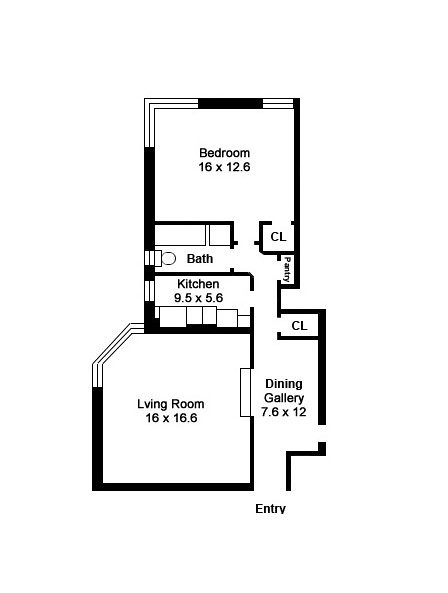This image depicts a detailed architectural blueprint of a one-bedroom apartment or condo. The layout starts with an entry point at the bottom, leading into a dining gallery measuring 7.6 by 12 feet, which has a closet situated at its back. To the left of the dining gallery is a spacious living room, measuring 16 by 16.6 feet. Behind the living room lies the kitchen, which is sized at 9.5 by 5.6 feet, with cabinets positioned at the bottom of the image.

Adjacent to the kitchen is the bathroom. The bathroom layout features a toilet on the left-hand side and a shower or bathtub above it. Directly across from the bathroom, there is a pantry. A hallway extends from the dining gallery, with a closet on the right and the kitchen on the left. The hallway continues, with the pantry on the right and the bathroom on the left, before slightly curving to the left, leading to the bedroom in the back.

The bedroom measures 16 by 12.6 feet and contains a closet situated in its front right corner. The bedroom features two windows: one on the back right wall and one in the top left corner. The living room also has a window where the top left corner is not squared off and instead features an angled cut.

The text on the blueprint is rendered in black, using a mix of uppercase and lowercase standard writing. Overall, the detailed layout illustrates a functional and compact one-bedroom apartment.